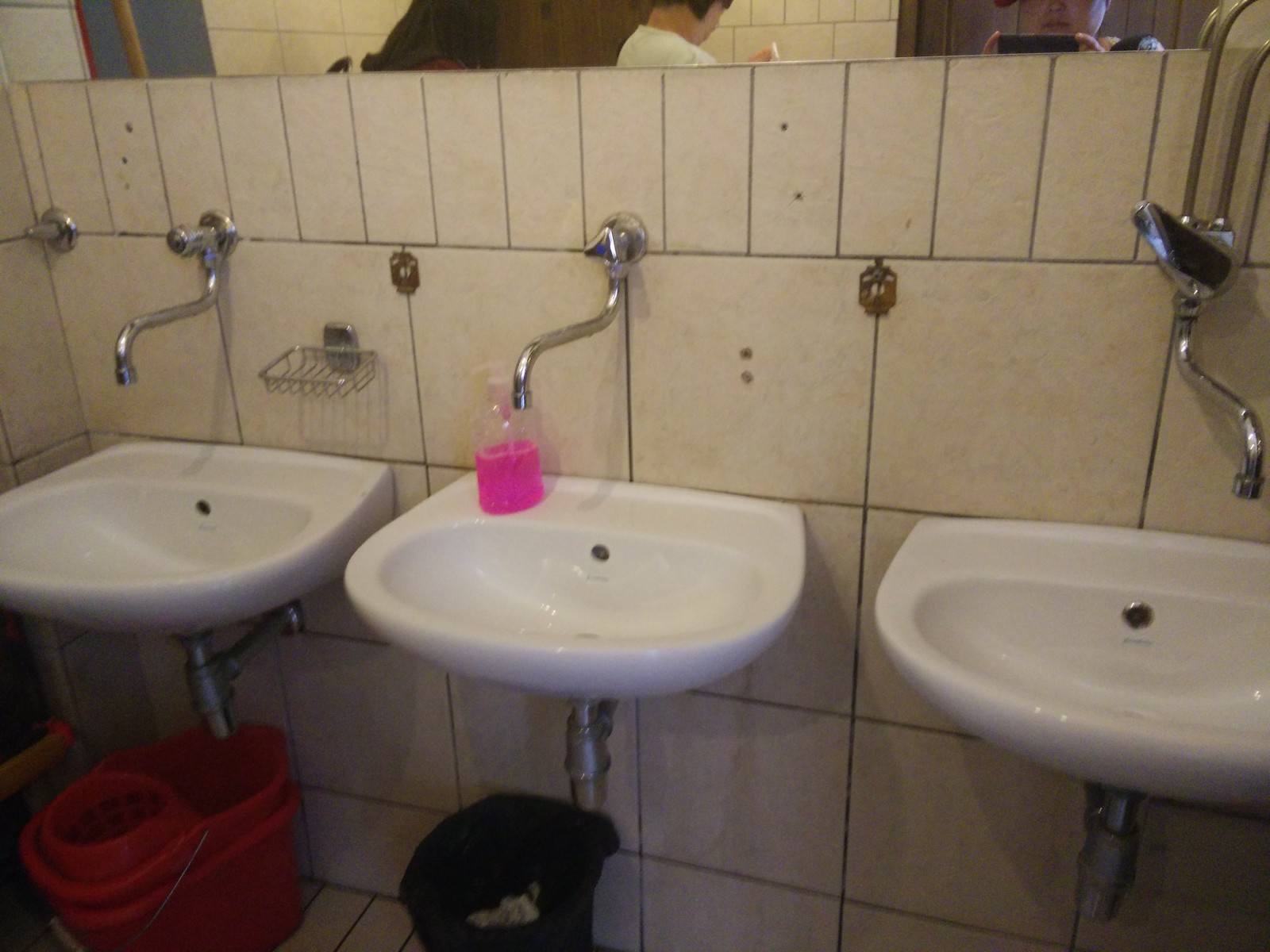This image depicts an old, public bathroom with three white sinks attached side by side to a dingy, beige-tiled wall. The tiles are square with a top row of vertical rectangles, giving a somewhat worn and unclean appearance. Each sink features a silver, S-shaped spigot mounted on the wall above it. There is a metal soap holder between the left and middle sinks, and the middle sink has a clear plastic bottle of bright pink liquid soap half-filled. 

Below the left sink, red buckets are placed on the floor, while a black bucket sits beneath the middle sink, possibly serving as a waste bin. The right sink is empty. A narrow strip of mirror above the sinks reflects two people: one holding a camera, presumably the photographer, and another woman with dark, straight hair and a white sweater, partially visible from the back.